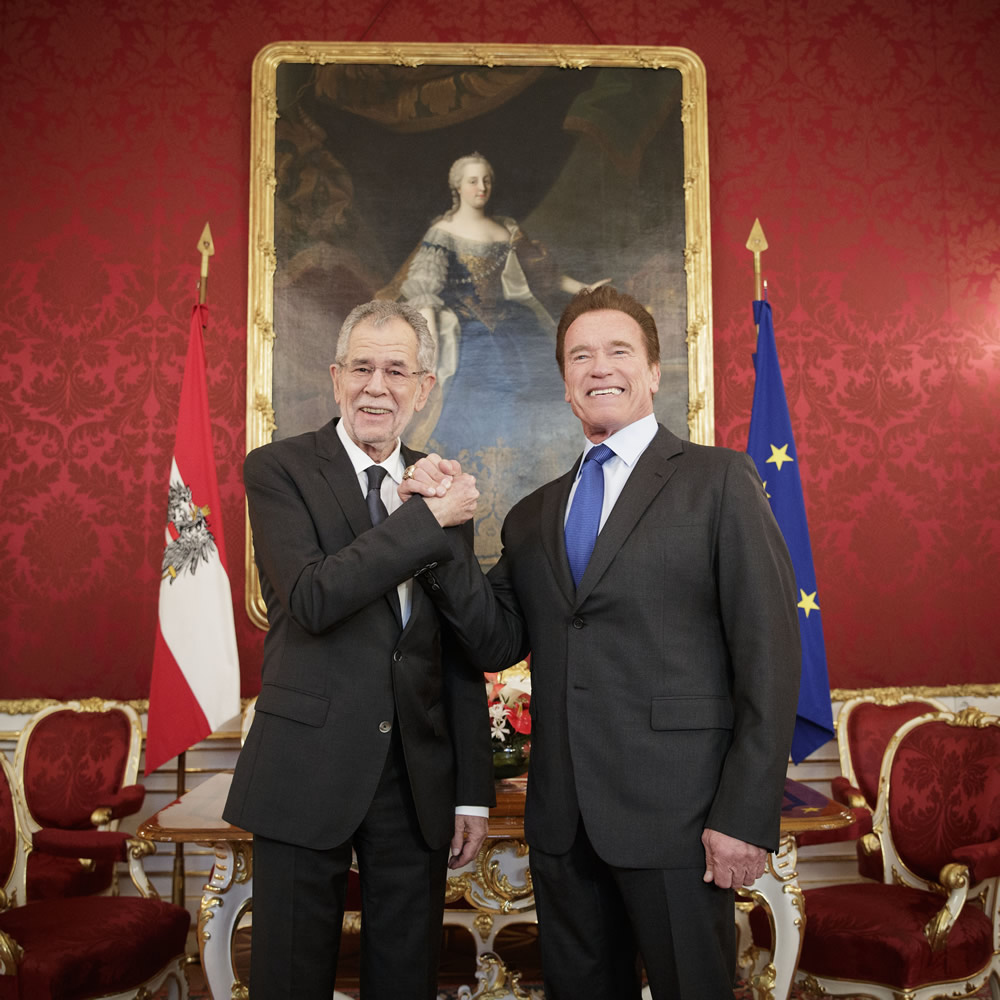In this image, two white men are standing side by side, shaking hands and smiling at the camera. Both are dressed in dark suits; the man on the right is wearing a blue tie, while the man on the left has a black tie and a white shirt. The setting appears to be a formal political or diplomatic room. Behind them, a large painting of a seated woman with a gold frame is centered on a red wall adorned with intricate designs. Flanking the painting are two flags: the Austrian flag, red and white with a design in the middle, and the European flag, blue with yellow stars. In front of the painting is an ornate white table with golden designs, topped by a bowl of flowers. Surrounding the table are four luxurious, red-cushioned chairs with white borders and gold accents. The rich red walls, elegant furniture, and symbolic flags suggest a setting of important cultural or political significance.